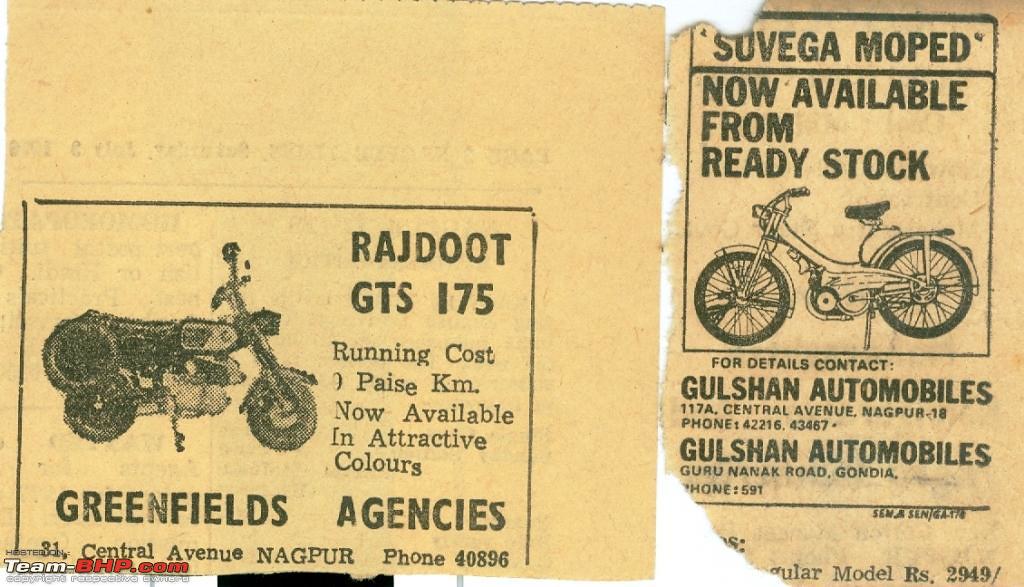This detailed photograph captures two vintage newspaper clippings, predominantly occupying the entire image space. The clippings, aged to a brownish hue, are juxtaposed side by side in a landscape orientation. On the left, the larger, square-shaped clipping advertises the Rajdhu GTS 175 motorcycle, featuring a black-and-white photograph of the bike. The text, albeit misaligned and faded, reads: "Rajdhu GTS 175. Running cost: Pays KM, now available in attractive colors. Greenfields Agencies, Central Avenue, Nagpur." The right clipping, resembling an old classified ad, showcases the Suvega Moped. This smaller advertisement includes a line-art illustration of the moped, accompanied by the text: "Suvega Moped, now available from Ready Stock. For details, contact Golshan Automobiles." The entire setting evokes a sense of nostalgia, with the tan, black, gray, and hints of red colors typical of aged print publications, and is further authenticated by a small logo at the bottom left reading "TeamBHP.com."